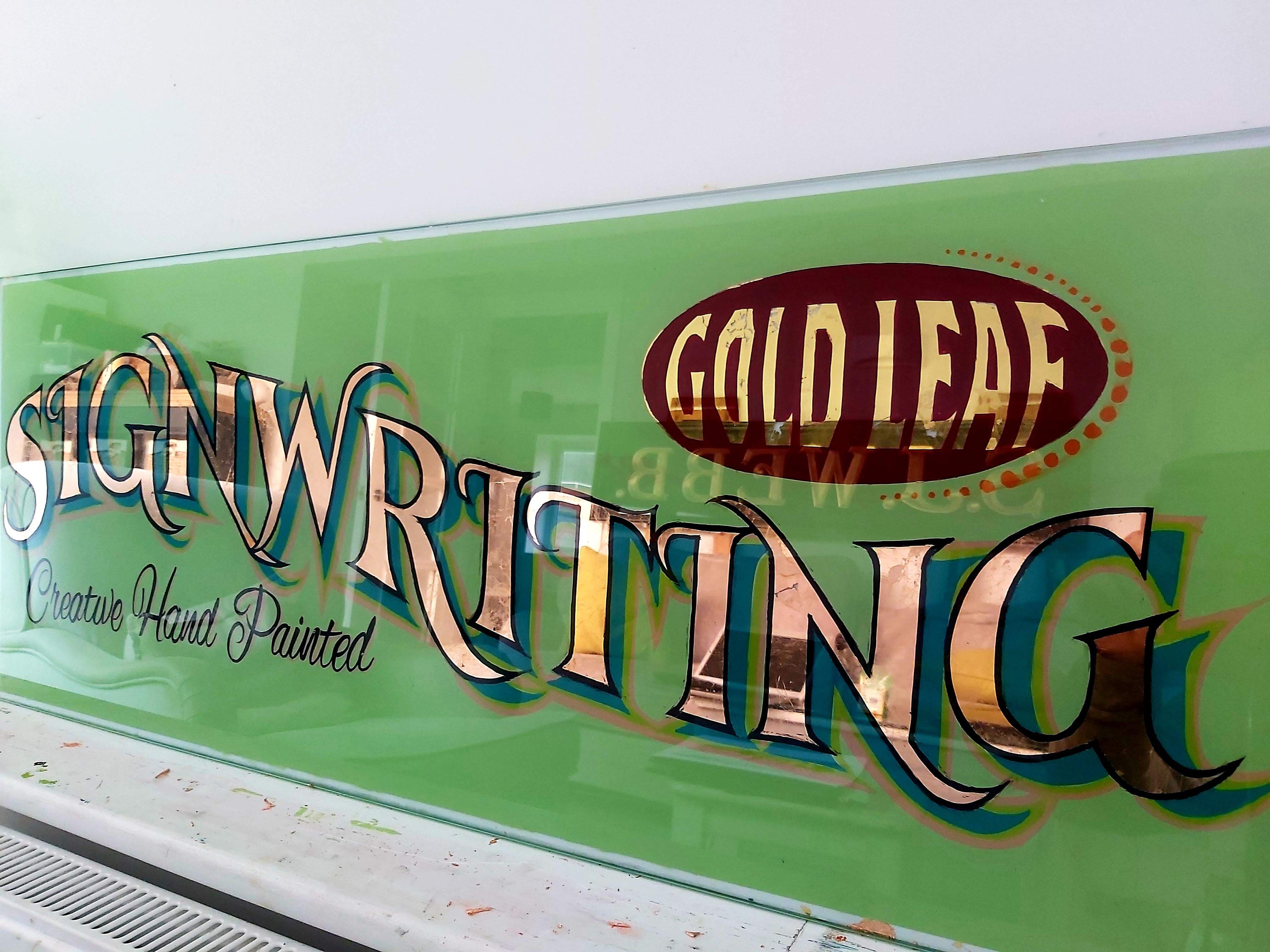The image depicts an indoor scene with white walls and a white ledge streaked with various colors. Atop the ledge is a large, glossy, rectangular glass sign with a transparent green background. The prominent feature of the sign is the phrase "SIGN WRITING" written in large gold capital letters, curving upward and then downward, with intricate blue and gold shadows. At the top right corner of the sign is a brown oval emblem with the words "GOLD LEAF" inscribed in gold, accompanied by red dots that arc around the right side of the oval. Beneath "SIGN WRITING," in elegant brown cursive, is the phrase "CREATIVE HAND PAINTED." The entire composition is reflective, indicating the sign's polished finish. In the foreground, there's a white metallic grate, possibly a vent, adding depth to the setting.